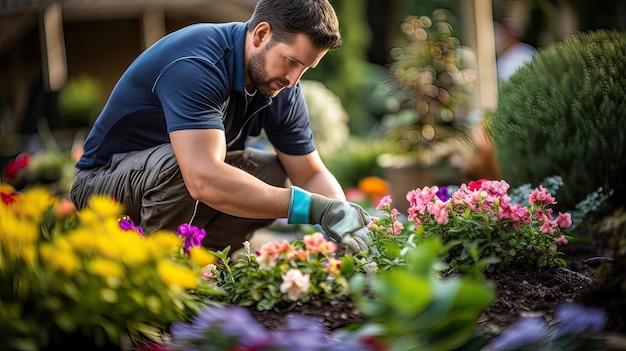The image depicts a Caucasian man, probably in his thirties, squatting and bending over in a flower bed, engaged in either planting or pruning flowers. He has short dark hair and a neatly groomed dark beard and mustache. He is wearing a snug, dark blue short-sleeved shirt, possibly with a zipper, and gray pants, complemented by gray and blue garden gloves with an aqua band. The man also sports a silver necklace. The flower bed is rich with colors, showcasing a variety of blossoms in pink, purple, peach, fuchsia, and red hues, with yellow flowers appearing blurred in the foreground. The soil in the flower bed is dark brown, surrounded by an abundance of green leaves. In the background, blurred scenery includes various green plants, a round bush to the right, and some potted plants, suggesting the setting could be a garden, perhaps outside someone's house or a garden center. Despite the man's meticulous appearance, more akin to a model, his pose and activity give the impression of genuine gardening work.